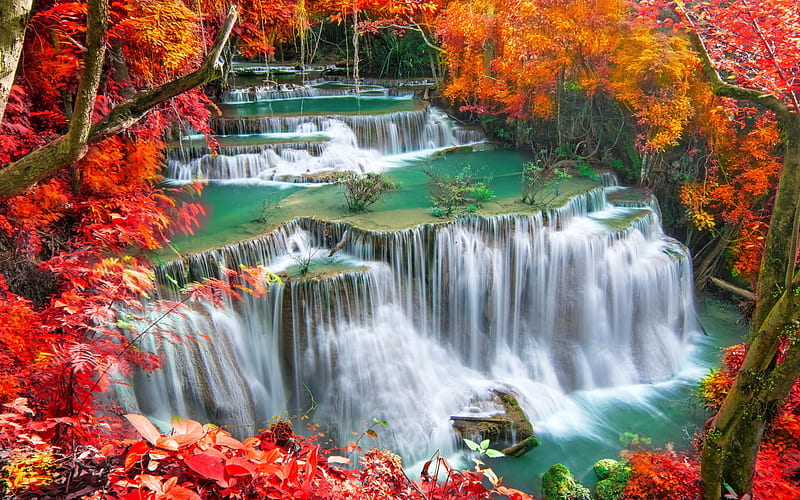This striking photograph captures a stunningly beautiful outdoor scene that almost appears AI-generated due to its surreal beauty. The main focus is a multipart waterfall system cascading into a bluish-green river. In the foreground, three prominent waterfalls flow energetically into the river, their white-capped currents contrasting vividly against the water's serene color. Above these falls, another smaller river can be seen feeding additional waterfalls, creating layers of rock formations between each cascade.

Alongside the waterfalls, there are rocks and scattered shrubs growing within the water, with some long reeds almost touching the rushing water, adding to the scene's complexity. The water features a blend of white and greenish-blue hues, with some calm areas reflecting the surrounding beauty.

Encircling the entire scene is a dense border of trees adorned in the vibrant colors of autumn, with leaves in varying shades of bright orange, red, and gold. Some trees appear mottled with moss, adding texture to the overall landscape. At the base of the waterfalls, large rocks emerge from the water, surrounded by an array of plant life. The entire image is framed with trees exhibiting peak fall foliage, enhancing the picturesque and serene autumn ambiance.